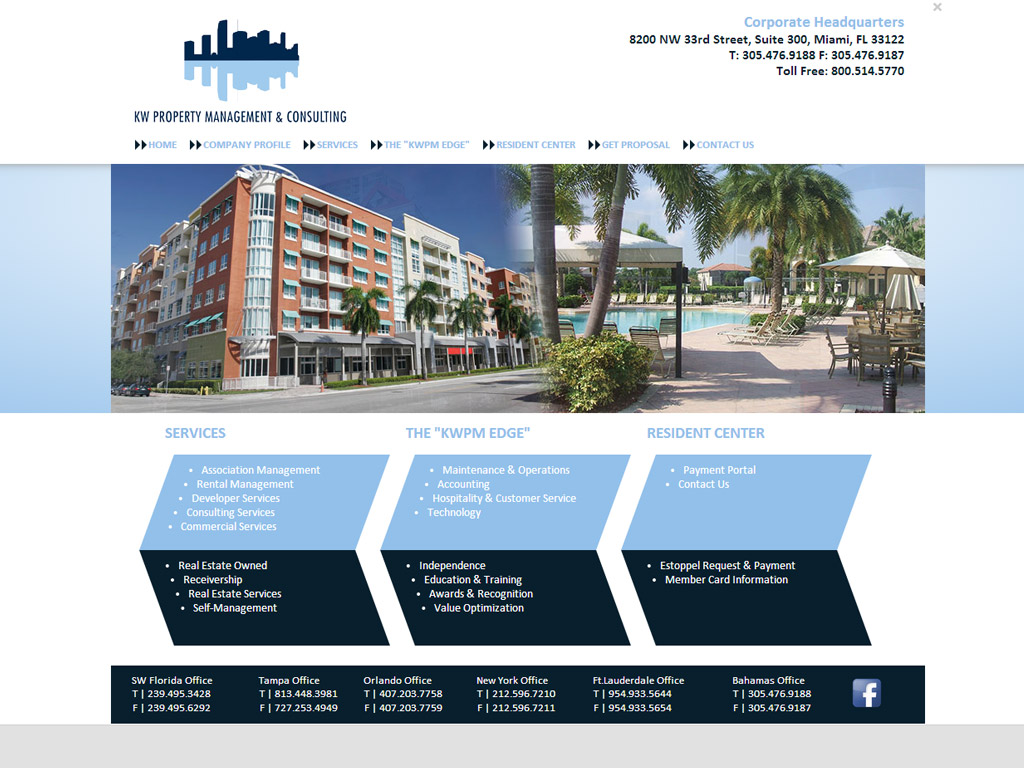This is a detailed description of a screenshot capturing a website from a computer monitor:

---

The image is a screenshot of a KW Property Management and Consulting website as viewed on a computer monitor. The top section of the website is a clean, all-white background featuring a dark silhouette of a skyscraper skyline. Below the skyline, a light blue reflection creates a mirror image of the buildings. 

In the upper right corner, there is a blue text box labeled "Corporate Headquarters," accompanied by the corporate address in black lettering. To the left of the skyscraper icon, the company name, "KW Property Management and Consulting," is prominently displayed in dark lettering.

A navigation bar runs across the top, consisting of several blue labels, each flanked by two small black right arrows. The labels, from left to right, read: Home, Company Profile, Services, the KW PM Edge, Resident Center, Get Proposal, and Contact Us.

Beneath this navigation menu, there's a high-quality image of a well-maintained, five or six-story brick building featuring a glass elevator located on a corner lot. The scene includes a sidewalk lined with palm trees on both sides and a clear blue sky overhead. On the right side, a large swimming pool can be seen behind the apartments, surrounded by cabanas.

Below this main image, a section features three arrow-shaped icons labeled in blue text. The first icon, labeled "Services," the middle one marked "The KW PM Edge," and the right-hand icon labeled "Resident Center." These sections are divided into a light blue top half and a black bottom half, with white text detailing various services and features. The "Services" section lists items such as Rental Management and Developer Services. The KW PM Edge section includes bullet points like Independence, Education, and Training. The Resident Center section lists features such as a Payment Portal and Contact Us.

At the bottom of the screenshot, a black banner stretches across the screen, detailing six different locations: Southwest Florida, Tampa, Orlando, New York, Fort Lauderdale, and the Bahamas. For each location, there are two contact numbers (presumably a phone and a fax), displayed in white lettering. A blue Facebook icon is positioned at the far right end of the banner.